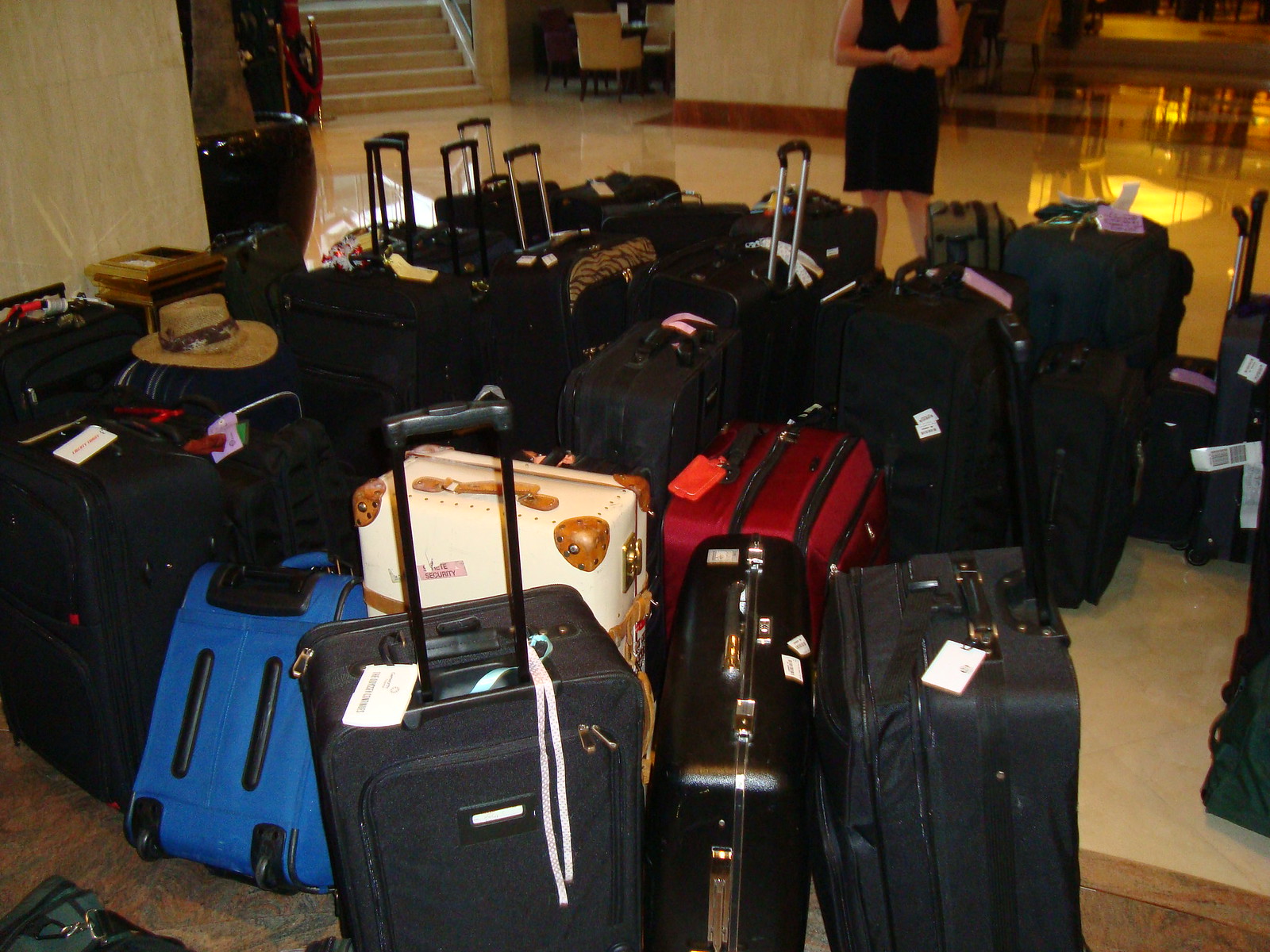In the lobby of an elegant, posh hotel, a large cluster of over 20 neatly standing suitcases is visible, most with their handles up, creating a structured pile. The majority of the luggage is black, but three distinctive pieces stand out: a red suitcase, a white suitcase with brown leather trim, and a small blue fabric carry-on. This assortment of luggage is situated on a section of the floor where plush, brown-and-orange paisley-patterned carpet meets a shiny, mirrored-type marble tile. An orange light casts a warm reflection on the tile at the top right corner, contrasting with a cooler white light reflecting on the left. In the background, stairs lead up to a cozy snug area with tables and chairs, adding to the grandeur of the hotel. Partially visible is a woman, seen from the knee down, dressed in a knee-length black skirt and bare arms, suggesting a sophisticated ambiance. The luggage suggests recent arrival, possibly by a coach, ready to be collected and taken to individual rooms. A hat rests atop one suitcase, and many have tags, hinting at the bustling activity typical of a high-end hotel reception area.